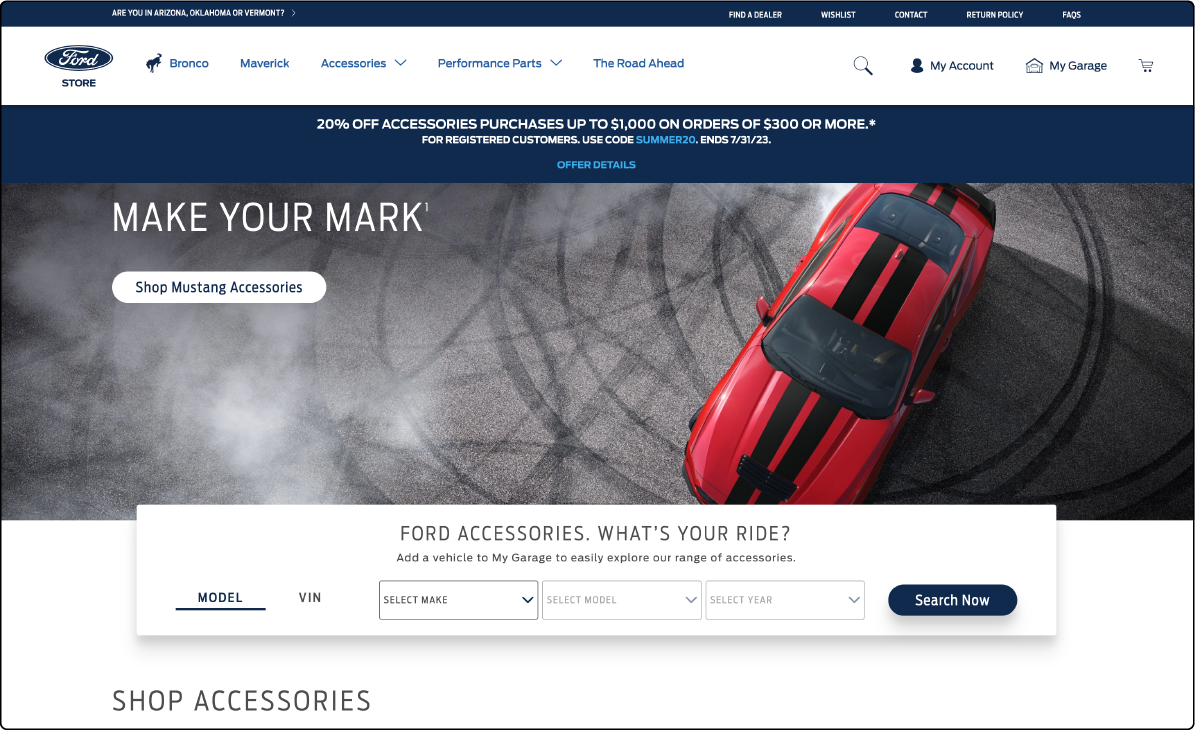This is a detailed and descriptive caption for the image of the Ford Store website's desktop version:

"Screenshot of the Ford Store website's desktop version. At the very top, a thin blue banner stretches across the page, featuring minuscule white text in the top left corner, while top right categories include: Find a Dealer, Wishlist, Contact, Return Policy, and FAQ. Just beneath this banner, a large white header prominently displays the Ford Store logo on the left. Adjacent to the logo, five categories are listed in small blue font: Bronco, Maverick, Accessories (with a drop-down menu), Performance Parts (with a drop-down menu), and The Road Ahead. On the page's top right, there are icons for Search, My Account, My Garage, and a shopping cart.

Directly below this header, a striking big blue banner proclaims: "20% off accessories purchases, up to $1,000 on orders of $300 or more." In a line of very small white text beneath this, it states: "For registered customers, use code SUMMER20 and 73123," with the code SUMMER20 highlighted in blue. At the bottom, light blue text reads: "Offer Details," centered in the bar.

Following this promotional banner is an expansive photo of a Ford Mustang performing donuts in a parking lot. Superimposed text on the right reads: "Make Your Mark" in large white letters. Below this, a white button prompts: "Shop Mustang Accessories." Located centrally at the photo's base, a large white box invites: "Ford Accessories," with the query: "What's Your Ride? Add a vehicle to My Garage to easily explore our range of accessories." At the bottom left of this box, 'Model' and 'VIN' are indicated, with 'Model' being selected and underlined in blue. In the center of this section, three drop-down menus are available labeled: Select Make, Select Model, Select Year. To the box's right, a prominent blue button labeled "Search Now" is visible. Further below on the left, partially visible gray text in all caps reads "Shop Accessories," though it is cropped off."